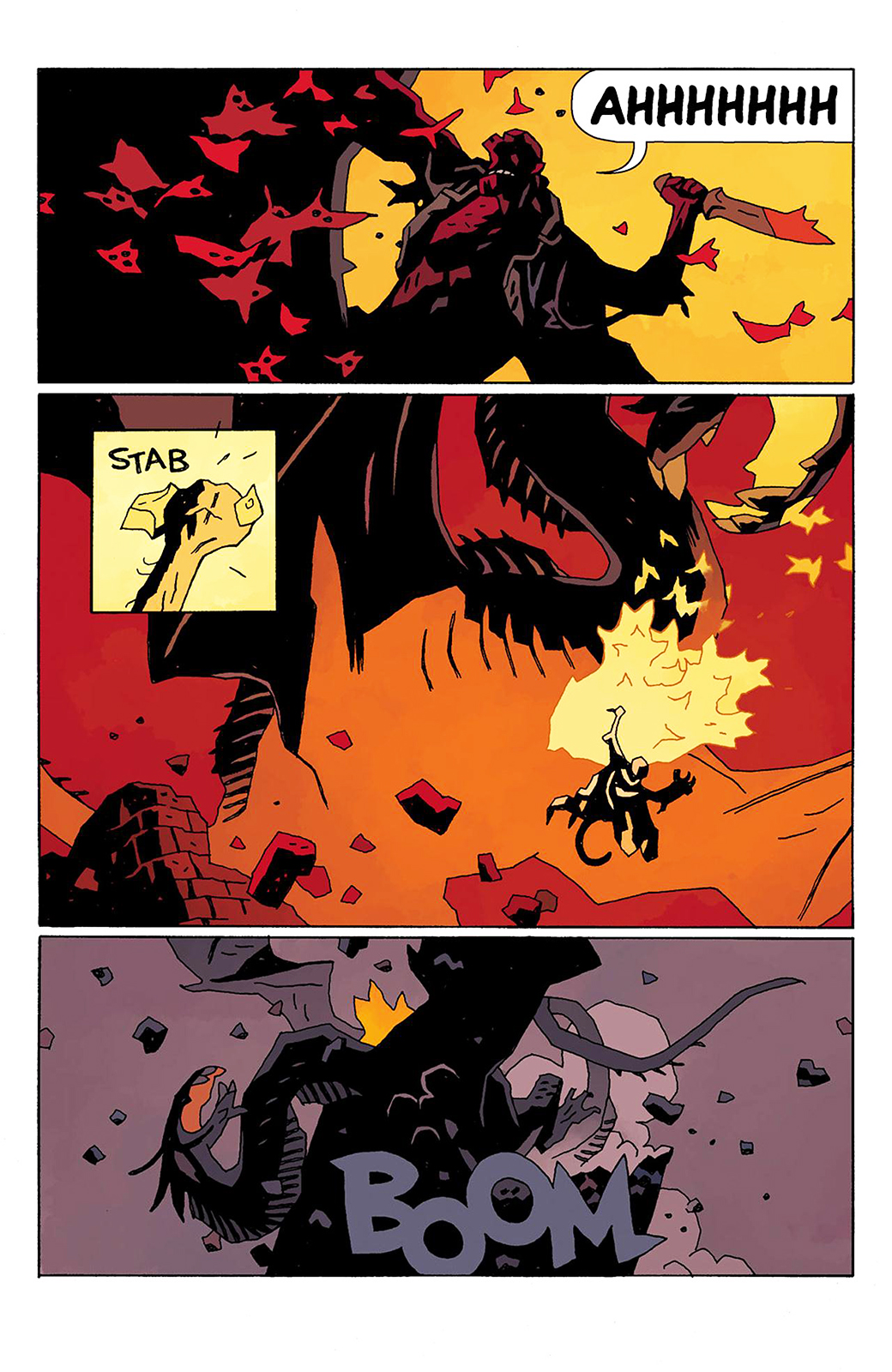This comic page features three vertically stacked panels depicting intense action scenes. In the top panel, Hellboy is partially silhouetted, holding a large, spike-tipped knife covered in red. He is poised to strike, with red, stylized, paper-like creatures flying around him, some punctured with holes. He exclaims "AH" in a word balloon. The background contrasts with black on the left and yellow on the right.

The middle panel includes a small inset labeled "Stab" with a yellow background and black text. Here, Hellboy is depicted stabbing a large dragon, with flames erupting around the point of impact. He seems to be holding onto the dragon amidst an orange and red-dominated background, suggesting intense heat and chaos.

In the bottom panel, the background transitions to purple as the dragon reels back in pain. Flames flicker from a crumbling structure, possibly a tower, and debris falls all around. The word "Boom" is displayed in a different shade of purple with offset letters, emphasizing the impact and destruction caused by Hellboy's attack.